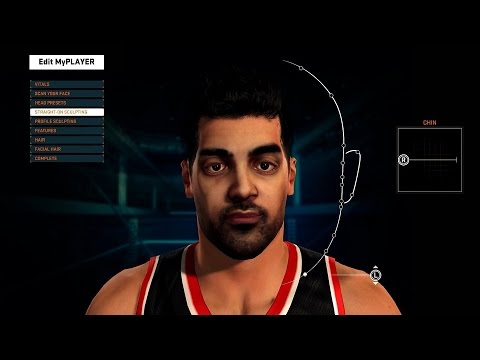A computer-generated image features a basketball player set against a flat, solid black background devoid of texture and dimension. The background is slightly accented with a series of faint grayish-green lines directly behind the player, adding a minimalistic touch. Dominating the center of the image is a male figure with black hair and tan skin, whose ethnic background is ambiguous but may suggest African-American heritage. His facial features include bushy eyebrows, a mustache, and a beard. He is clad in a black, sleeveless jersey accented with red and white trim around the v-neck and shoulder area. To the right of the player, text reads "Chin," accompanied by a white box with a horizontal line and a white circle containing an indistinguishable letter, possibly an "A" or "R." On the left side, an "Edit My Player" box is visible, with various options displayed in orange text against a lighter black or gray background. One of these options is highlighted in white, indicating a selection for editing the player's attributes.